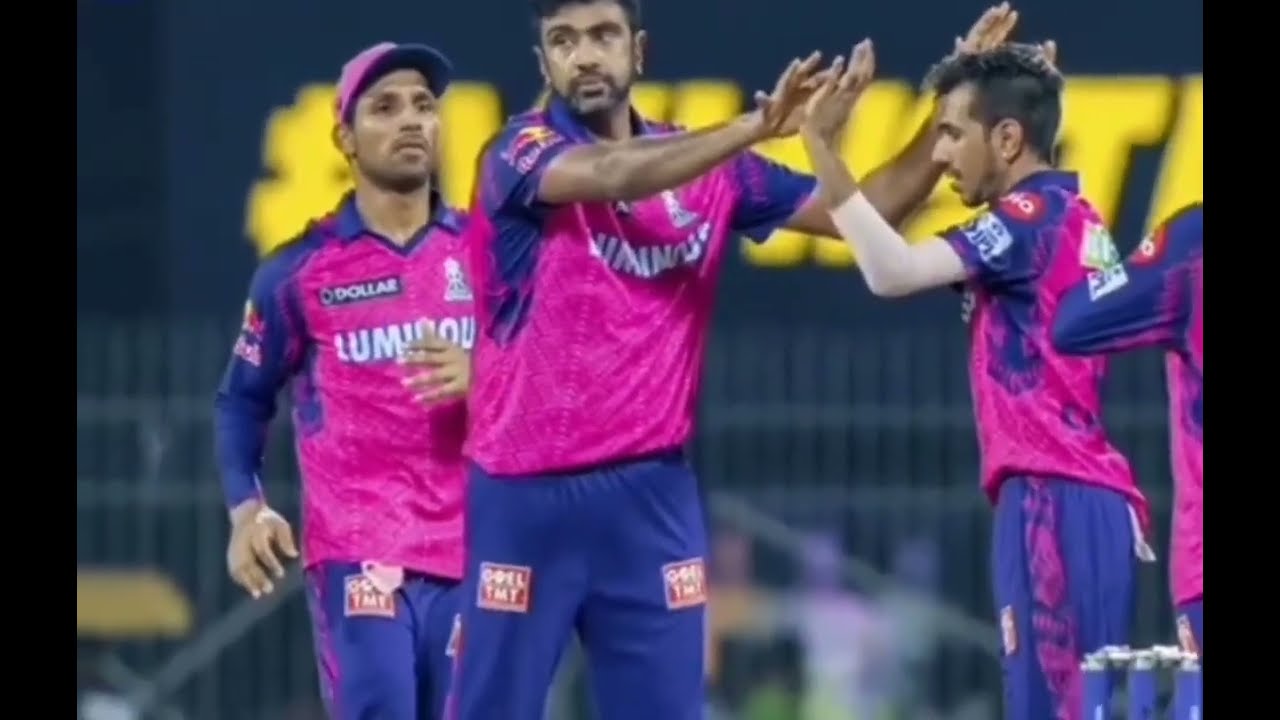This color photograph, seemingly captured from a screen with black letterbox bars framing the top and bottom, showcases an outdoor scene featuring four athletes in a sports arena. The players are donning short-sleeve, collared uniforms that blend pink and blue hues, with blue sleeves and pants. The central focus is on two athletes giving enthusiastic high-fives with both hands, while a third player, slightly blurred, approaches from behind wearing a matching ball cap. The fourth player's elbow and back are visible at the right edge of the frame. All the athletes have short brown hair and brown skin. The jerseys display the team name, partially obscured, as "L-U-M-I O-U," with a prominent logo or patch reading "Dauer" on the upper left chest. In the background, a wire fence and a yellow sign with illegible text can be seen amidst an indistinct, possibly crowded, backdrop.